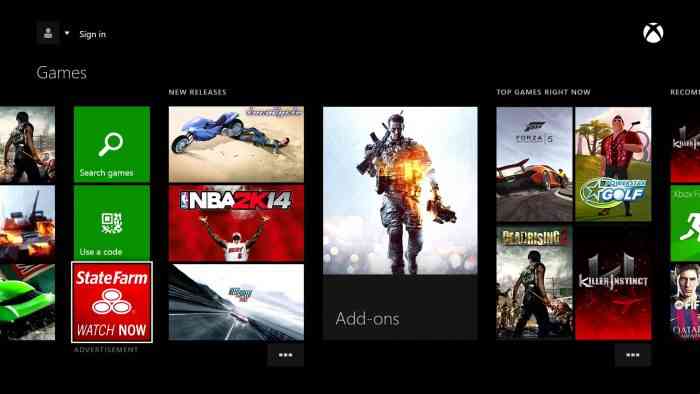A screenshot displays what appears to be the Microsoft Store interface, showcasing a selection of games available for purchase. Prominently featured are titles like "NBA 2K14" and "Tiger Woods PGA Tour." Several game icons are partially visible but are not easily identifiable; one of them seemingly belongs to "Forza Motorsport 5." The background of the interface is predominantly black, lending a sleek and modern appearance. In the top right corner, an Xbox logo is clearly visible, indicating that the store might also serve as the Xbox Store. The interface includes a "Sign in" option, suggesting that users can log in for a more personalized experience.